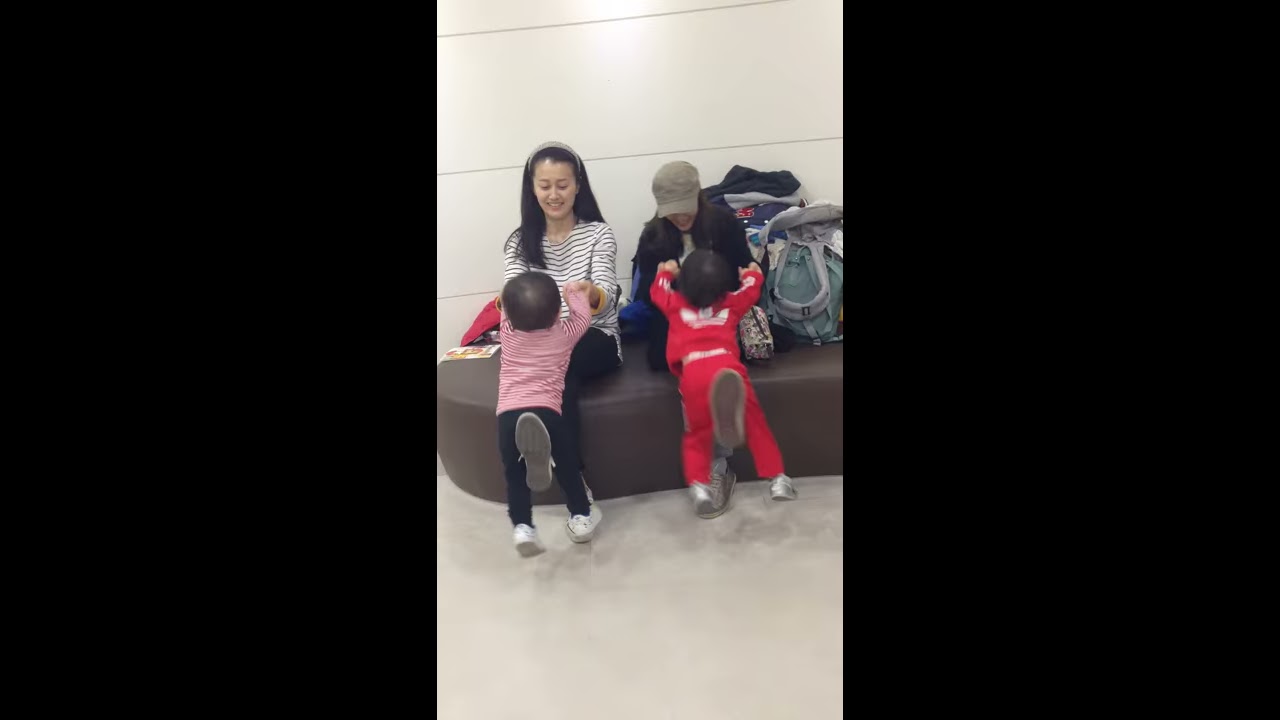In this image, we observe a family likely waiting for their next flight in an airport waiting area. The scene features two females, possibly a mother and her teenage daughter, sitting on a backless bench with brown cushions. The mother, situated on the left, has long dark hair and is wearing a striped shirt. She's playfully engaging with a toddler in a red and white striped long-sleeve shirt, black pants, and white tennis shoes, who is straddling her leg.

To her right, her teenage daughter, dressed in a dark jacket and a gray baseball cap, is similarly engaging with another toddler. This toddler, attired in a red Adidas sweatsuit and white tennis shoes, is also straddling the teenager's leg. Several bags and luggage are placed on the right side of the scene, indicating that the family is likely waiting for transportation. The setting appears to be an airport, with white and plastic-like walls and carpeting.